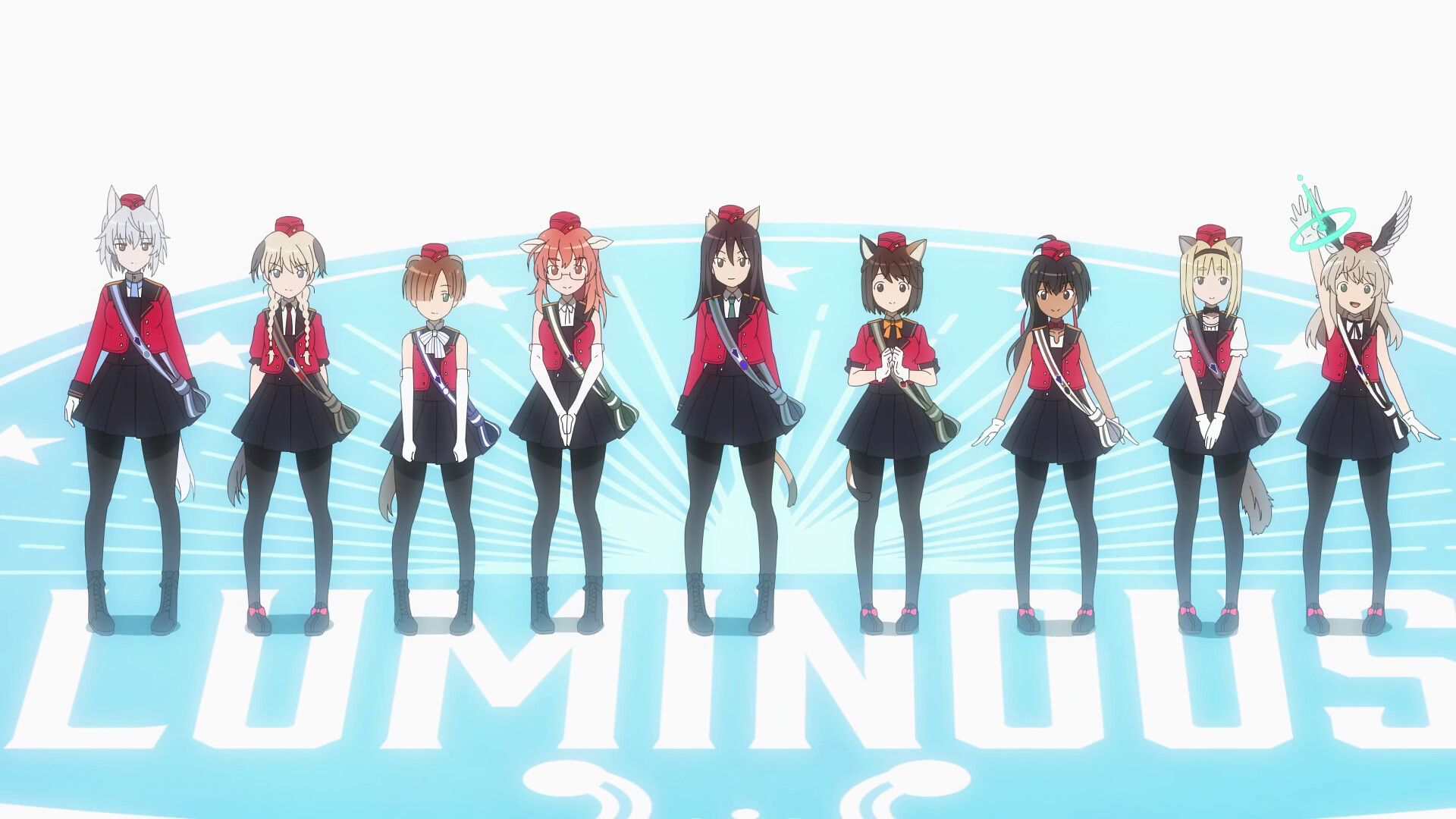This is a detailed cartoon anime-style image featuring nine female characters standing on a light blue logo with white capital letters spelling "Luminous." The logo sits prominently at the bottom of the image, set against a gray background, and appears to have radial lines and stars emanating from it. All nine characters are attired in coordinated outfits consisting of red and black jackets or shirts, black mini skirts, and black tights, with black shoes adorned with red bows or red socks. 

Notably, the characters exhibit a variety of hairstyles: some have gray hair, others have blonde hair styled in braids, and some sport short brown hair. Many of them appear to have cat ears, with at least six or seven displaying this feature, and they wear small, red, circular hats resembling hockey pucks. Accessories and props such as weapons are visible on a few, adding to their distinct appearances. The character on the far right stands out with her hand raised and a turquoise circle around it, from which something is protruding. Additionally, she has wings attached to her back. This image captures a vibrant and classic manga aesthetic.